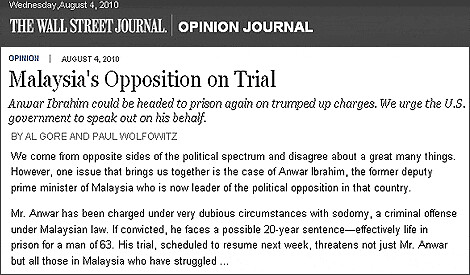This image is a clipping from the Wall Street Journal's opinion section, dated Wednesday, August 4th, 2010. At the top, within a black box, it reads "Wall Street Journal Opinion Journal". Below, it repeats the date, "August 4th, 2010", followed by the headline, "Malaysia's Opposition on Trial". The main text, authored by Al Gore and Paul Wolfowitz, states: "Anwar Ibrahim could be headed to prison again on trumped-up charges. We urge the U.S. government to speak out on his behalf." The authors note their differing political backgrounds but unite in support of Anwar Ibrahim, the former Deputy Prime Minister of Malaysia and current opposition leader. He faces charges of sodomy under dubious circumstances, a criminal offense in Malaysia. If convicted, he could face a 20-year sentence, effectively a life sentence for a 63-year-old. The trial is set to resume next week and poses a threat not only to Anwar but to all who have struggled in Malaysia. The text is printed in black font on a white background.